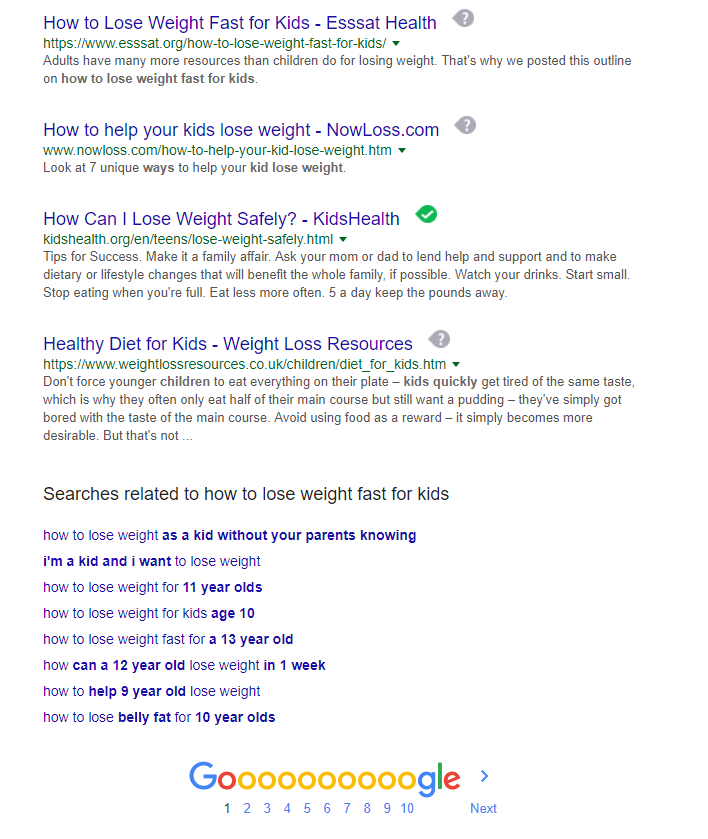This detailed descriptive caption conveys the information clearly:

---

The image is a screenshot of a Google search results page. At the bottom of the image, the Google logo is prominently displayed with the letters "G" and "O" in blue and red, respectively, followed by a series of yellow "O"s, and ending with "G", "L", and "E" in various colors. Below the logo, numbered page navigation links from 1 to 10, along with a blue arrow for the next page, are visible.

The search query is related to weight loss for children. The top result, highlighted in blue text, reads, "How to Lose Weight Fast for Kids - Asset Health," followed by a snippet of information. Below it, the second result is titled, "How to Help Your Kids Lose Weight - nowloss.com." The third result, "How Can I Lose Weight Safely - Kids Health," is accompanied by a green checkmark on the right side. Further down, there is another result titled "Healthy Diet for Kids - Weight Loss Resources."

At the bottom of the screenshot, a section labeled "Searches related to how to lose weight fast for kids" lists other related search queries. These include "how to lose weight as a kid without your parents knowing," "I'm a kid and I want to lose weight," "how to lose weight for 11-year-olds," and "how to lose weight for kids age 10," among others.

This image captures a Google search page focused on inquiries about children's weight loss and related health information.